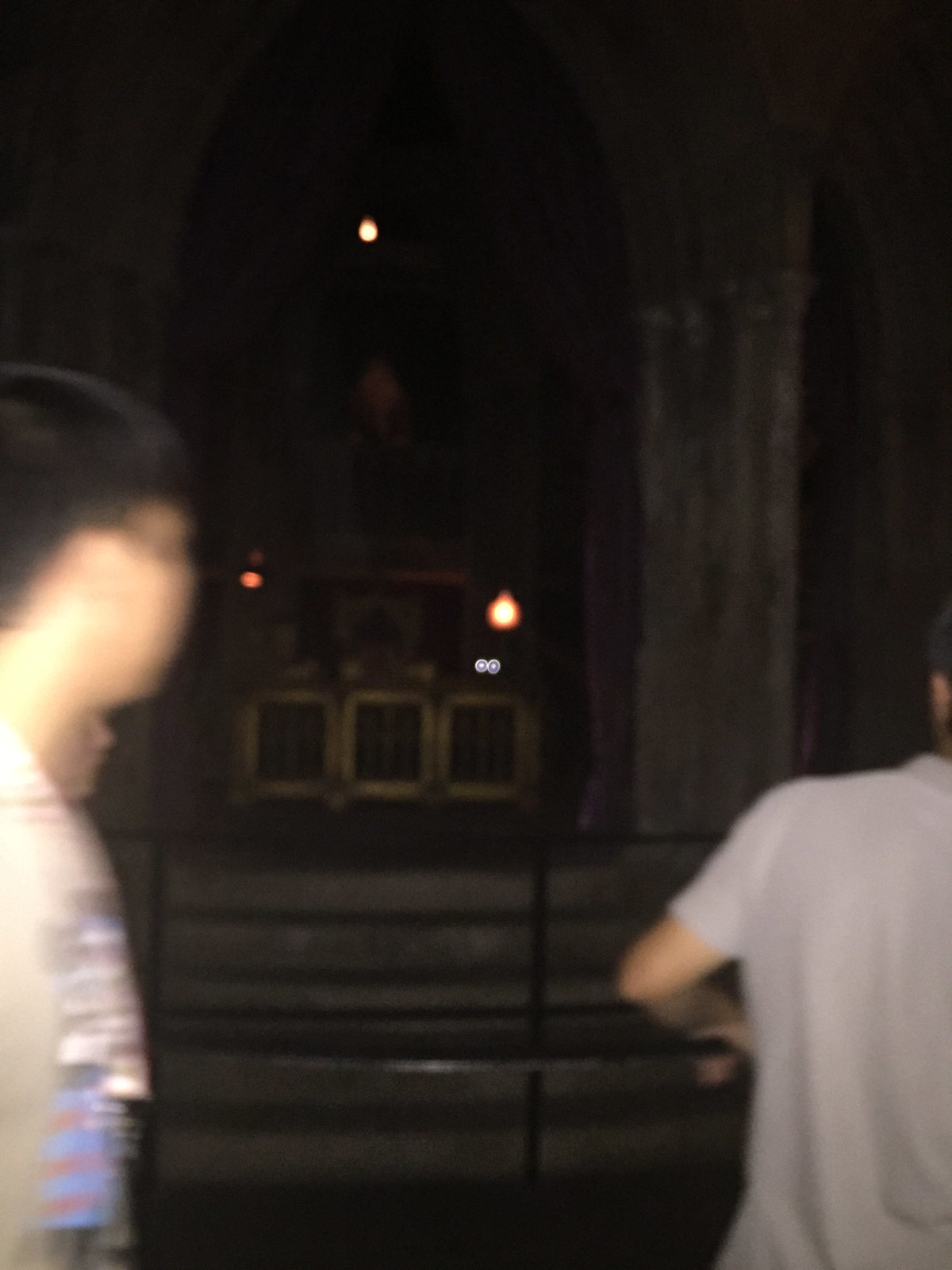This image is a blurry, dark photograph taken inside what appears to be an old-fashioned church or possibly a themed attraction designed to mimic such an environment. At the center of the image, there is a set of concrete steps that lead up to dark concrete pillars. Between two of these pillars, an opening reveals three small, golden-faced box structures that resemble ornate cages. These are topped by a countertop adorned with small bowls and a picture. Just above, there seems to be a small, dimly lit balcony. Lights on either side of the space do little to illuminate it, adding to the gloom. In the foreground, there are three blurry figures, likely children, behind a black metal railing that serves as a barrier. The overall scene exudes an old-world, possibly sacred atmosphere, embellished with gold trimmings and what appears to be church symbols, adding to the impression that it could be a tomb or a religious setting.